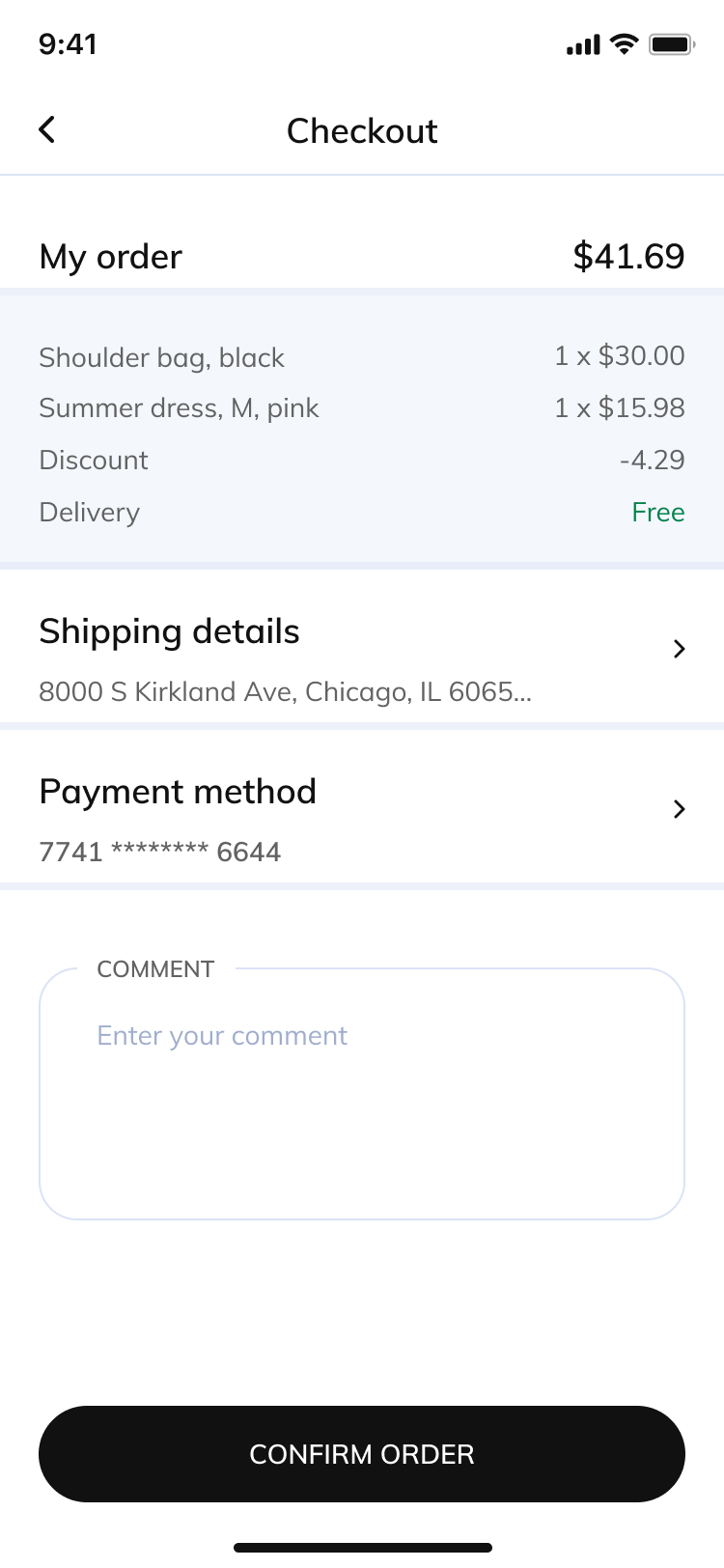This is an image of a purchase screen, specifically a screenshot of a phone browser displaying the checkout page. At the top left corner, the time is shown as 9:41. In the top right corner, there are several icons including a full signal bar, a Wi-Fi icon, and a fully charged battery icon displayed horizontally. 

Across the center header, the word "Checkout" is prominently displayed, accompanied by a back arrow icon to its left. Below this header, two columns are presented. The column on the left starts with "My Order" while the column on the right shows the total amount: $41.69.

Underneath this section, a gray box continues the two-column format, detailing the items in the order. The left column lists:
- Shoulder Bag
- Black Summer Dress, M, Pink
- Discount
- Delivery

Correspondingly, the right column lists:
- 1x $30.00
- 1x $15.98
- -$4.29 (negative amount)
- Free

A section for shipping details follows, displaying the address: "8000 S Kirkland Avenue, Chicago, Illinois 6065..." with an arrow to the right for more details.

Below the shipping details, another box shows the payment method as "7741 **** 6644" with an arrow to the right for further information.

Further down is a text box labeled "Comment", with placeholder text prompting "Enter your comment".

At the very bottom of the screen, there's a black button with white text that reads "Confirm Order". This area also features a horizontal scroll bar indicating additional content can be viewed if scrolled.

The overall layout is clean and detailed, providing all necessary information for completing a purchase.